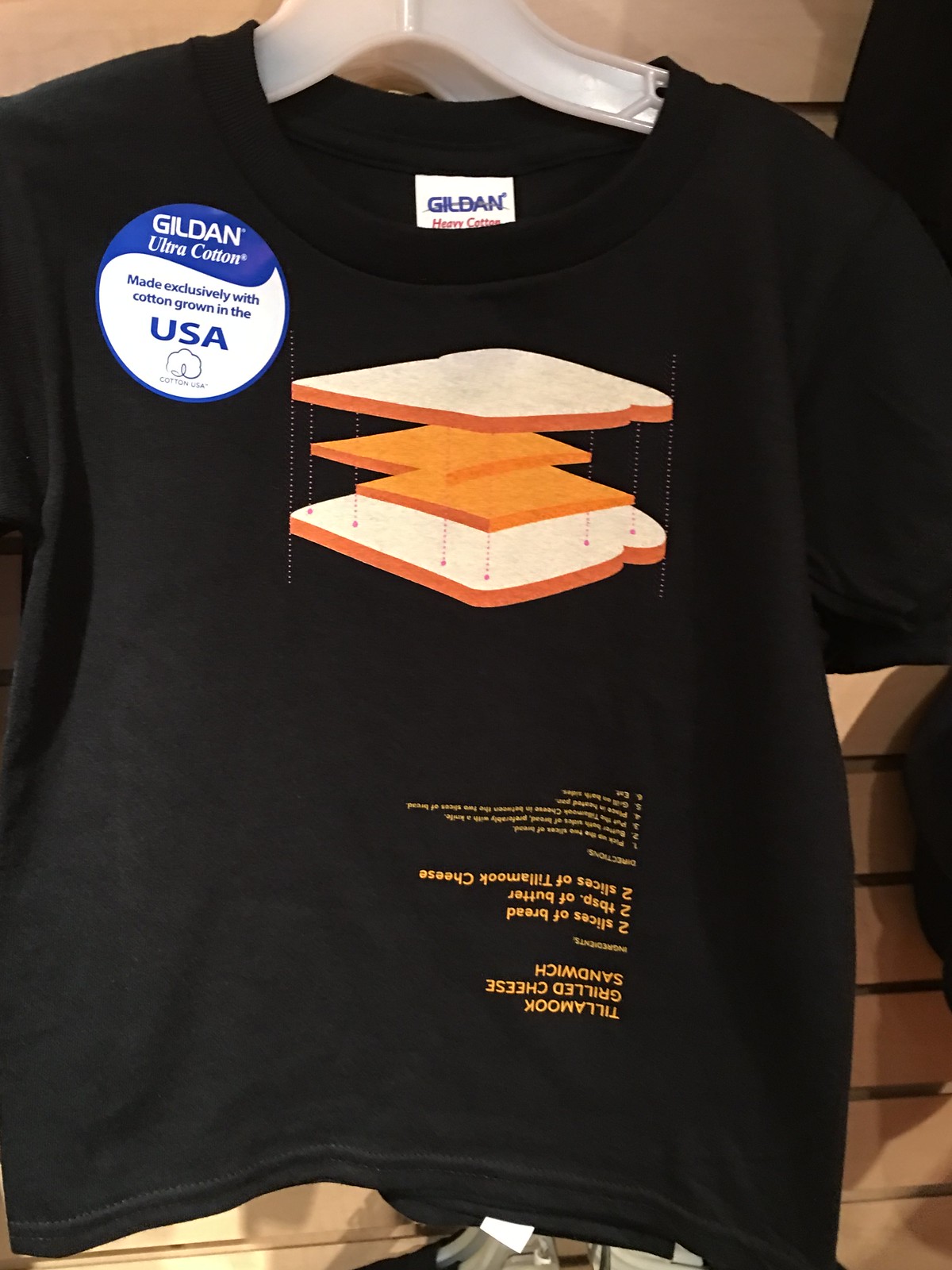A new Gildan Ultra Cotton t-shirt is displayed prominently in a store. This black t-shirt, adorned with an official Gildan tag, proudly states it is made in the USA. The shirt features a quirky design: at the top, there is a white and blue graphic of a cheese sandwich consisting of two slices of white bread and a layer of yellow cheese, separated by little spaces to clearly depict each element. The text accompanying the image, possibly detailing the sandwich ingredients or instructions, is printed upside down with blue lettering. The shirt hangs on a white hanger, which is placed on a stand with slots designed specifically to hold hangers. It is surrounded by other black t-shirts, blending into the retail environment, yet standing out with its unique design and vibrant print.